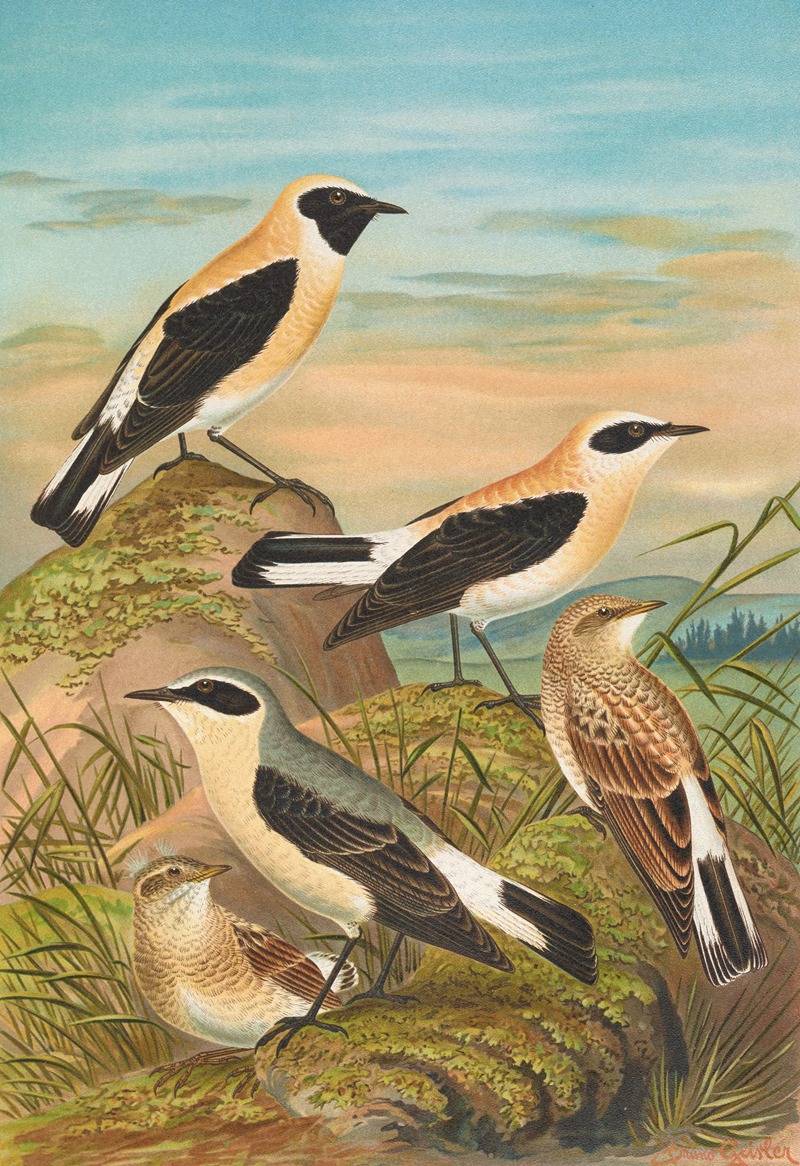This rectangular painting, taller than it is wide, captures a serene outdoor scene with a backdrop of a blue and brown-gray sky. Sandy-colored clouds linger overhead, enhancing the tranquil setting. The foreground features a rocky outcropping with patches of moss and tufts of long grass strewn between the stones. Perched on these rocks are five distinct birds, each detailed with intricate care.

The bird at the highest point on a little rock sports a striking look with its black face and throat, a brownish-orange body, black wings, and a tail patterned in black and white. Next to it, another bird of similar size lacks the black throat but otherwise shares similar coloration. Below them, a slightly smaller bird displays a gray head and back instead of the brown, but it retains the black wings and a black and white tail. The remaining two birds, situated lower and to the left, differ from the others, exhibiting a more speckled brown and white plumage, reminiscent of a sparrow, and also have the signature black and white tails.

This composition of colors and textures against the sky and rocky terrain provides a harmonious glimpse into the natural world, capturing the varying appearances and subtle differences among the birds.